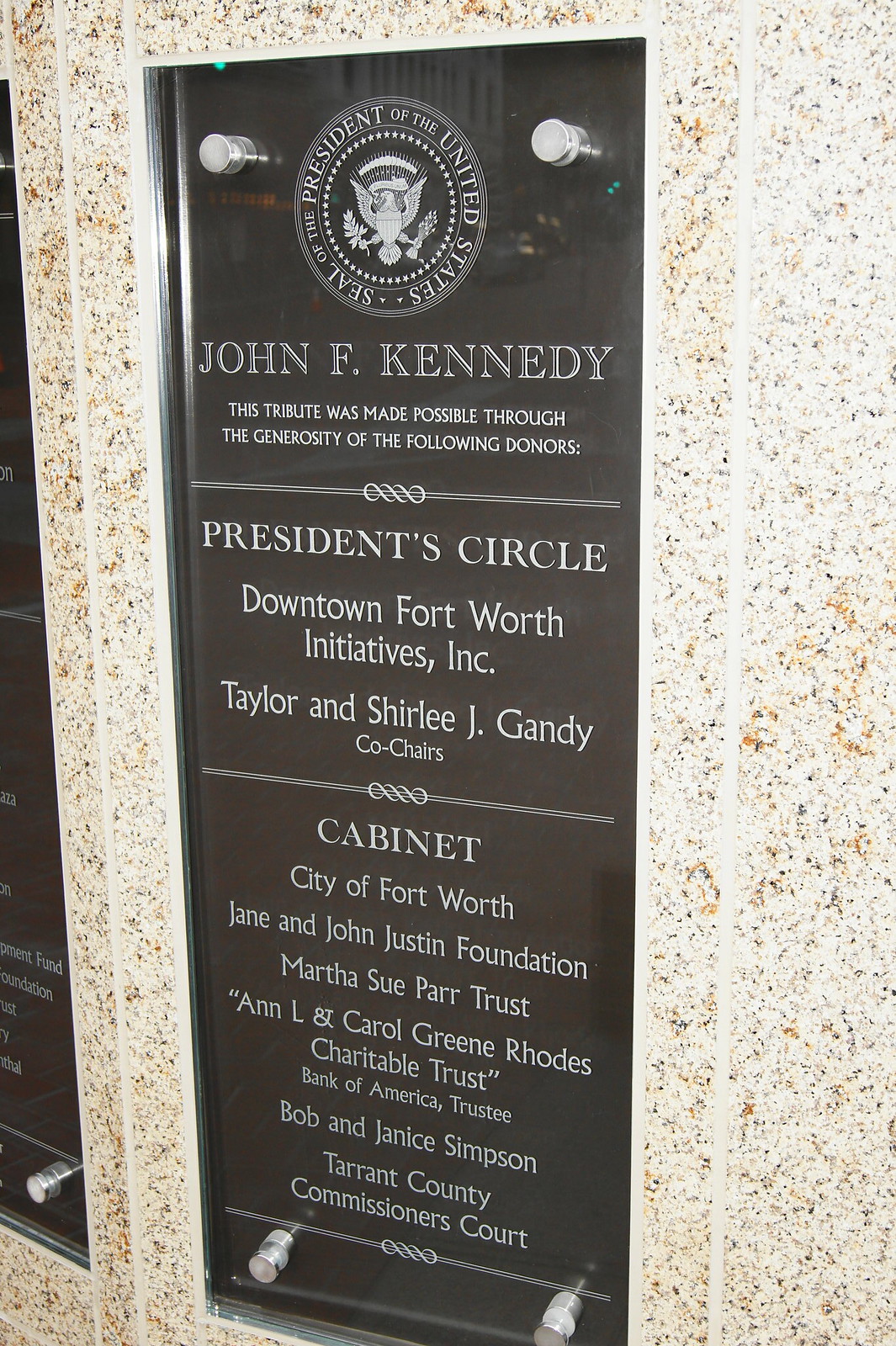The image is a color photograph in portrait orientation, showcasing a rectangular, dark-colored tribute plaque mounted on a beige speckled granite wall. At the top of the plaque is the seal of the President of the United States in white, followed by "John F. Kennedy" in large white letters. Beneath this, in smaller text, it reads "This tribute was made possible through the generosity of the following donors," followed by a double white line. Below that, in bold, it lists "President's Circle" and then details the contributors: "Downtown Fort Worth Initiatives, Inc., Taylor and Shirley J. Gandy, co-chairs," followed by another white line. The text continues with "CABINET," the "City of Fort Worth," and several other donors including "Jane and John Justin Foundation, Martha Sue Parr Trust, Anne L. and Carol Green Rhodes Charitable Trust, Bank of America Trustee, Bob and Janice Simpson, and the Tarrant County Commissioners Court," with each name on a new line. The plaque, a tribute to President John F. Kennedy, signifies the collaborative effort and generosity of various donors in honoring his legacy.